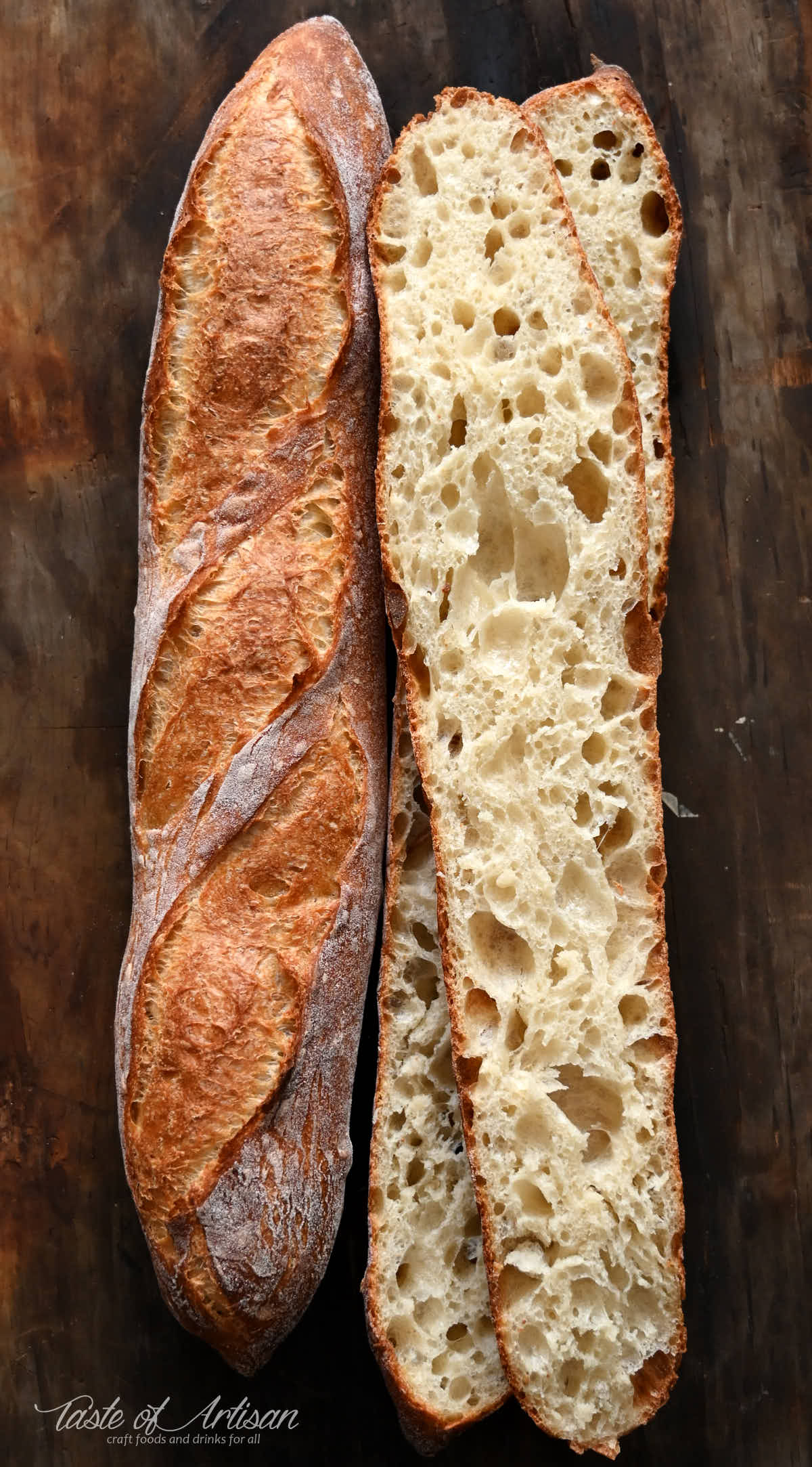The image showcases two artisan loaves of bread artfully laid out on a weathered dark-brown wooden table. The loaf on the left, which is uncut and elongated like a traditional baguette, features a light brown, flour-dusted crust with three diagonal slashes revealing a reddish-brown, fluffy interior. The similar-sized loaf on the right has been sliced cleanly down the center, displaying its airy, cream-colored interior with visible air pockets. The slices are positioned with one slightly offset atop the other, providing a glimpse of the loaf beneath. In the bottom left corner, the white cursive text reads "Taste of Artisan," with the subtitle "craft foods and drinks for all" in smaller, regular font.